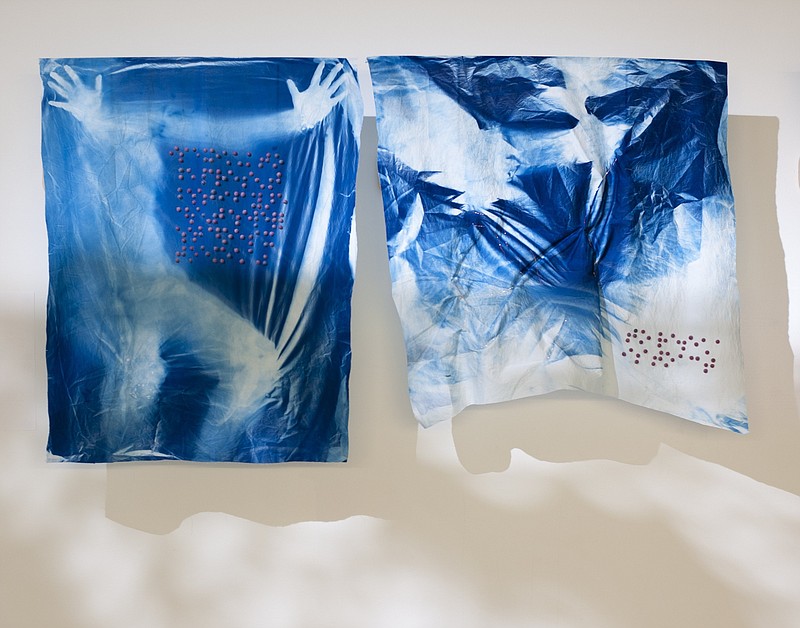In this image, there are two hand-dyed fabric artworks displayed on a table. Both pieces predominantly feature shades of blue, white, and gray, with muted spots of color. The artwork on the left has a central design created by placing hands on the fabric and spraying dye around them, resulting in white handprints against a blue background. It also contains some muted round dots in diverse colors like pink, yellow, and blue. Additionally, there is braille text at the top-center of this piece. The second artwork on the right showcases white silhouettes resembling birds against a blue backdrop. The bottom right corner of this piece has less dye, appearing mostly white, with brown round dots scattered throughout. This piece also features braille text positioned at the bottom right. The remaining areas of both pieces have gray and white hues, and the overall setting suggests these are artistic, possibly gallery-displayed, creations.